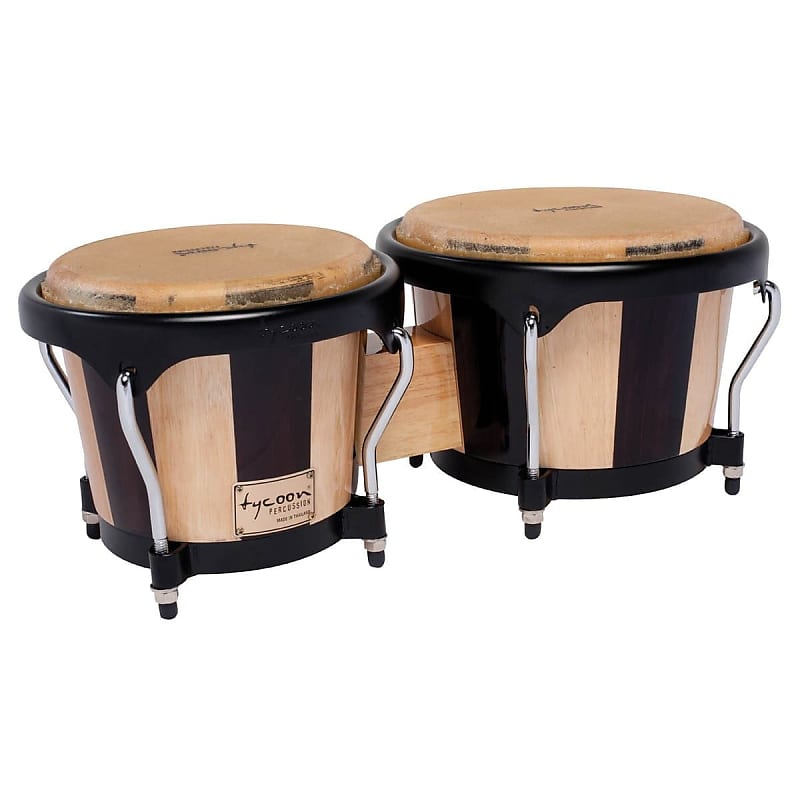This image showcases a pair of interconnected hand drums, commonly known as bongo drums, prominently displayed against a plain white background. Crafted primarily from wood, the drums feature a tan to light brown coloration, complemented by black trim around the edges and supporting structures. Notably, the drums display chrome accents along the sides and robust steel legs extending from the drumheads to the bases, ensuring stability. Each drum is linked by a sturdy piece of green wood. 

The left drum bears the logo of Tycoon Percussion, presented as a beige badge with the word 'Tycoon' written in a distinctive, lowercase signature style, and 'Percussion' printed underneath. Signs of wear and use are visible on the tops of the drumheads, suggesting that these drums have seen some use and may be second-hand items. The photograph captures a direct, eye-level view, emphasizing the craftsmanship and details of the drums within a minimalistic setup that focuses solely on the instruments.